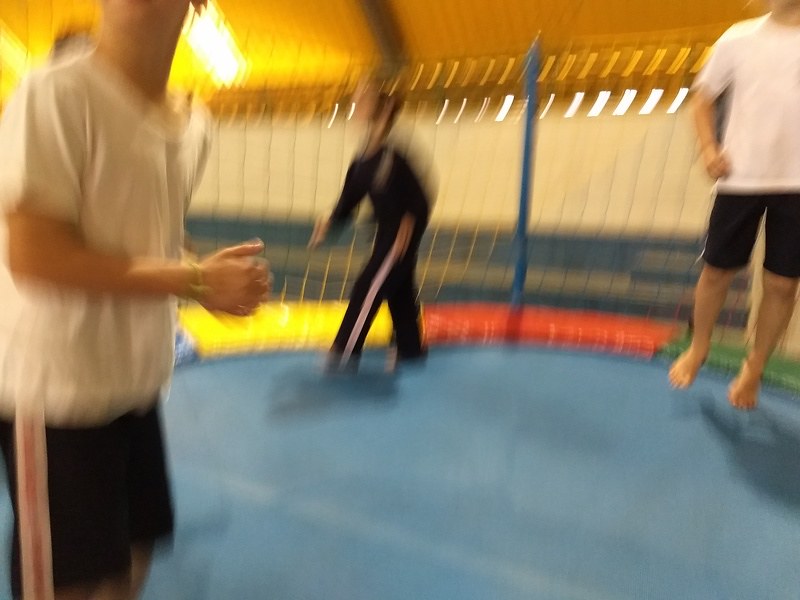In the image, a group of individuals are energetically bouncing on a blue trampoline. On the left side, a person dressed in a white shirt and black shorts, adorned with white and red stripes along the sides, is in mid-jump. To the right, another individual, also in a white shirt and black shorts, joins them. Among the jumpers, one is clad in an all-black outfit featuring a striking white stripe with a hint of red.

Surrounding the trampoline is a colorful border padded for safety, displaying hues of yellow, red, and green. In the background, a rope with blue caps can be seen. Overhead, the rooftop slopes downward and is painted yellow, with a lighting fixture partially visible in the top-left corner, casting shadows across the scene. The backdrop showcases a white wall under a blue section, providing contrast and framing the lively trampoline activity.